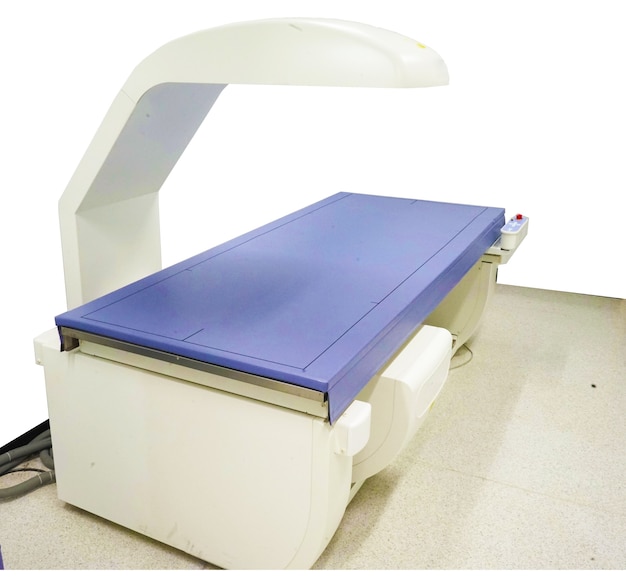This image depicts a detailed medical examination setup centered around a modern scanning machine. Dominating the room with beige and white walls, the machine features a blue examination bed atop a white base, designed for patients to lie on for body scans. An overhead device, which is the scanning apparatus, hovers above a part of the bed, presumably to conduct thorough scans of the patient's body. On the right side of the machine, there is a red button alongside several controls, indicating functionalities for operating the device. Notably, the gray-tiled floor is visible, with power cables placed on the left. This sophisticated setup reflects the advanced technology employed in medical diagnostics.